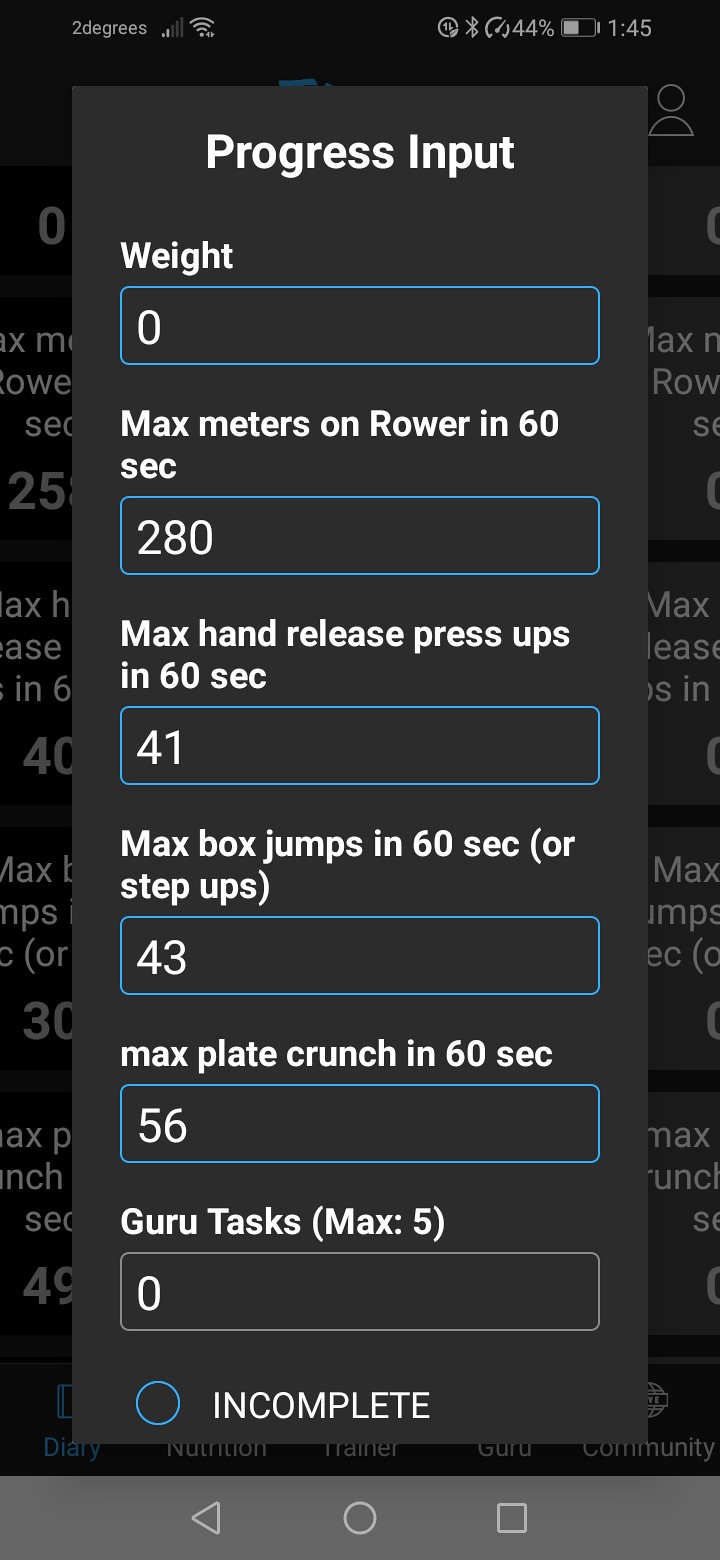The image is a screenshot from a mobile device, predominantly featuring a black background with white text. At the top of the screen, there are common phone status icons, including a Wi-Fi signal, battery percentage at 44%, and the time showing 1:45. Positioned in the center of the screen is a prominent white rectangular overlay titled "Progress Input." This overlay lists several performance metrics with corresponding input boxes, all presented in blue. The metrics are as follows: "Wait" with an entry of '0', "Max meters on rower in 60 seconds" with '280', "Max hand release press-ups in 60 seconds" showing '41', "Max box jumps or step-ups in 60 seconds" with '43', and "Max plate crunch in 60 seconds" with '56'. Additionally, there is a section labeled "Guru tasks" where "Max" is set to '5' but currently displays '0'. Below these metrics, a blue circle indicates the status as "Incomplete."